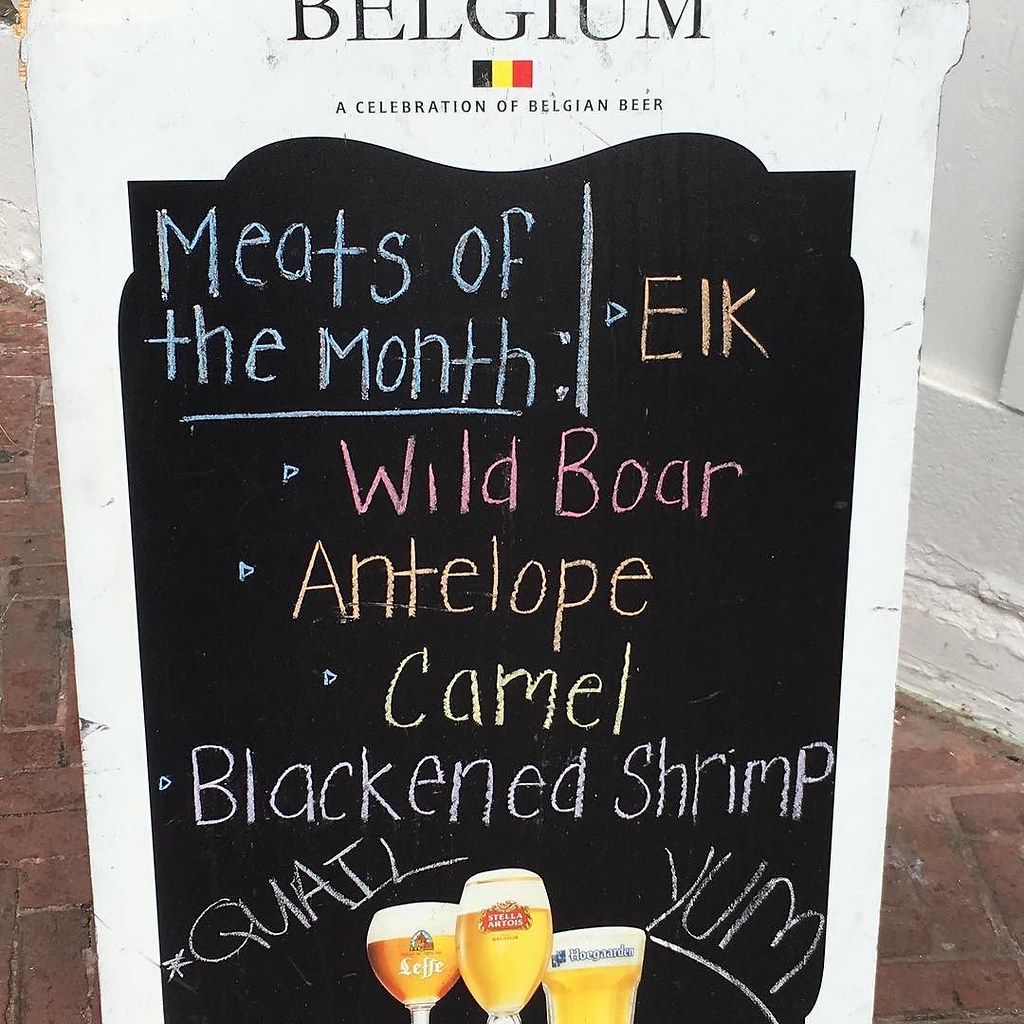The image features a foldout sidewalk advertising chalkboard sign, prominently displaying a vibrant and enticing message. At the top of the sign, the word "Belgium" is written in colorful chalk, heralding a celebration of Belgian beer. Accompanying this text is a depiction of the tricolored Belgian flag, adding a touch of national pride. Below, in blue-green chalk, the sign announces "Meats of the Month," listing an intriguing selection of exotic meats in green chalk: elk, wild boar, antelope, camel, blackened shrimp, and quail. An enthusiastic "Yum!" is inscribed at the bottom right corner. The lower part of the sign showcases the emblems and logos of several beers, alongside illustrations of three different styles of pilsner glasses. The glass on the far left is more akin to a wine glass, whereas the center and right glasses are distinctly pilsner style—tall and thin, designed to enhance the flavor by reducing foam. The board rests on a herringbone-patterned cobblestone brick sidewalk, adding to the rustic charm. In the background, an old building with layers of worn paint hints at a rich history, completing the picturesque scene.